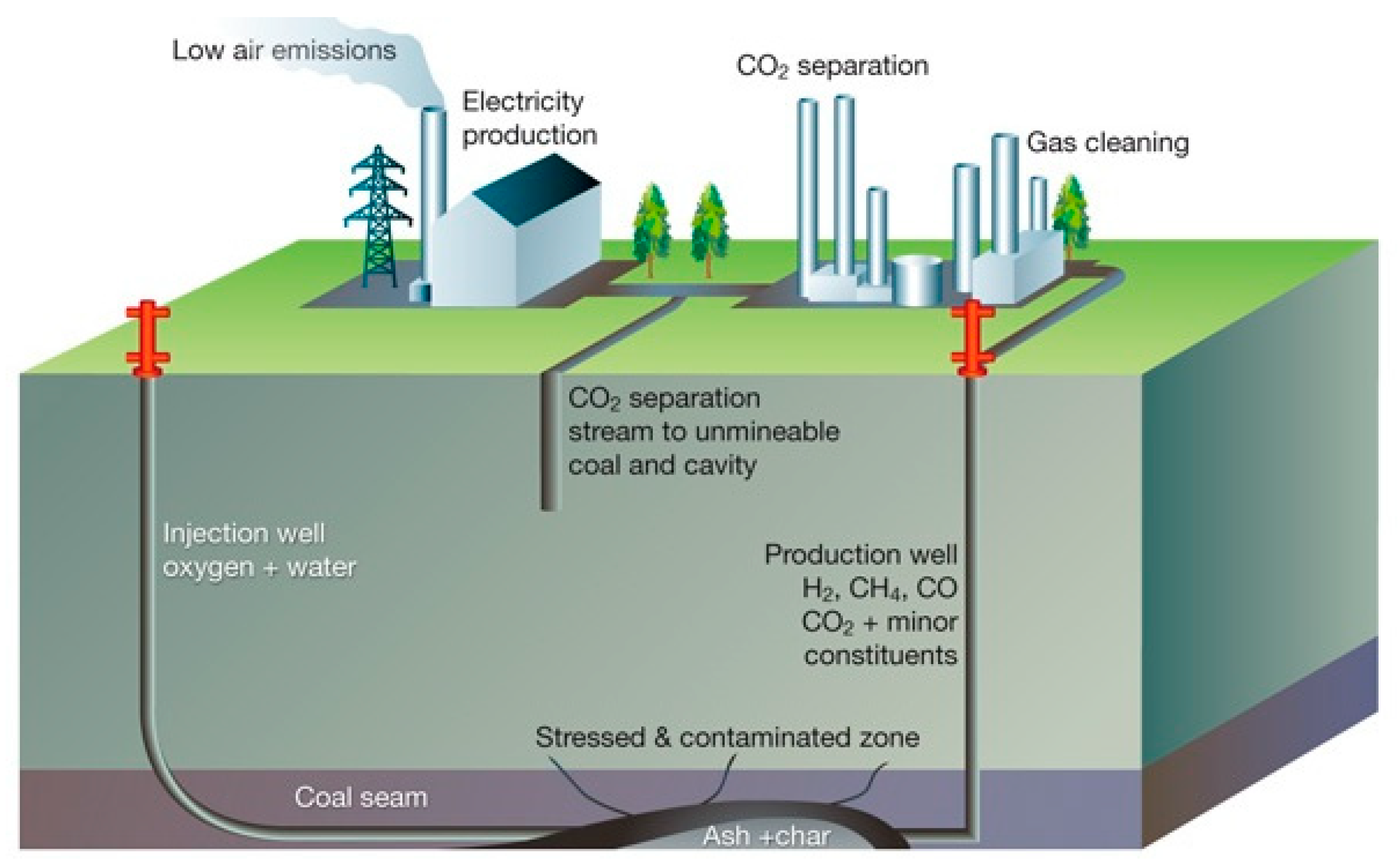The illustration depicts a detailed cross-sectional diagram of an eco-friendly energy production system with low air emissions, set atop a verdant landscape. On the surface, a green lawn is dotted with trees and buildings, including a house and an electrical tower. Central to the diagram are various smokestacks of different heights, emitting cleaned gas post CO2 separation. 

Marked in gray, the diagram shows an underground CO2 separation stream directing towards an unmineable coal cavity. Further right, a red production well, indicated by gray tubing, descends into the earth, channeling gases like H2, CH4, CO, CO2, along with minor constituents, down to a small purple coal seam. Another red injection well on the left is connected with oxygen and water tubes that also delve into the coal seam.

The subsurface areas include labeled zones like a stressed and contaminated section, illustrated with pointers leading to an ashen and char layer beneath. This comprehensive diagram emphasizes advanced technologies for electricity production and emissions control, integrating both above-ground and subterranean components in a highly detailed manner.